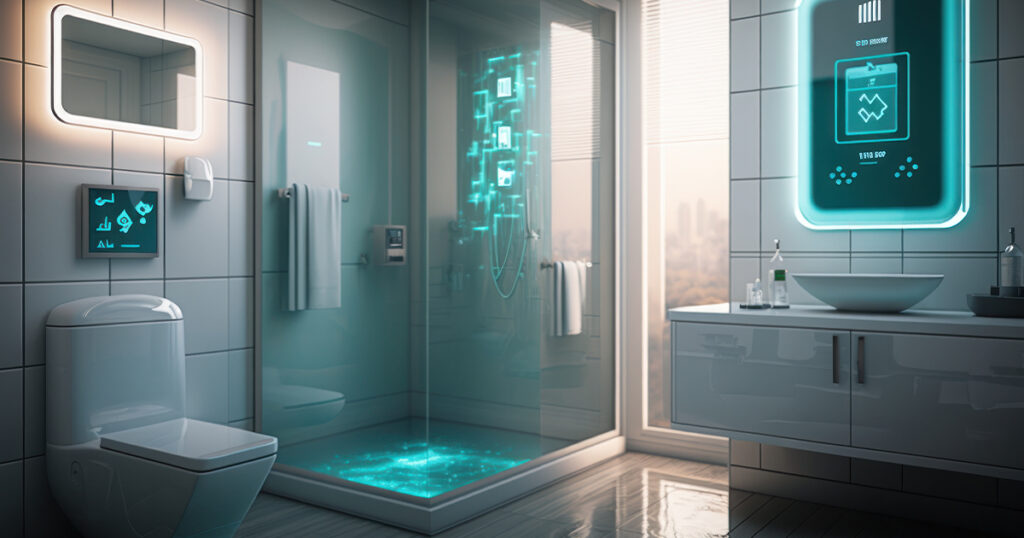This image showcases an ultra-modern, futuristic bathroom where sleek design meets technology. The walls are pristine white, adorned with white tiles that enhance the clean, minimalist aesthetic. The floor features a luxurious white marble look. On the left-hand side, a unique square-lidded toilet is situated below a high-tech digital monitor with various interactive logos, presumably for functions like flushing and bidet. Directly below this display, the toilet's design is seamlessly integrated into the wall with no visible flush mechanism.

Further to the right, a standing glass shower faces the camera, revealing an electric blue floor and a towel hanging from a rack on the left inside wall. The open shower lacks a traditional enclosure, adding to the bathroom's contemporary vibe. Adjacent to the shower, a full-length window with a white border allows natural light to flood the space.

To the right of the window, a gray wall features a floating, blue-bordered digitized control panel, resembling a futuristic cell phone. Below this panel, a sleek white sink with two outward-opening doors is positioned, atop it a basin-style bowl sink. Accompanying the sink are small jars, contributing additional modern touches. Above, an electronically lit mirror with a neon blue border adds a vibrant accent, enhancing the room's technologically advanced atmosphere. The recurring neon blue elements throughout the bathroom create a cohesive, futuristic theme.